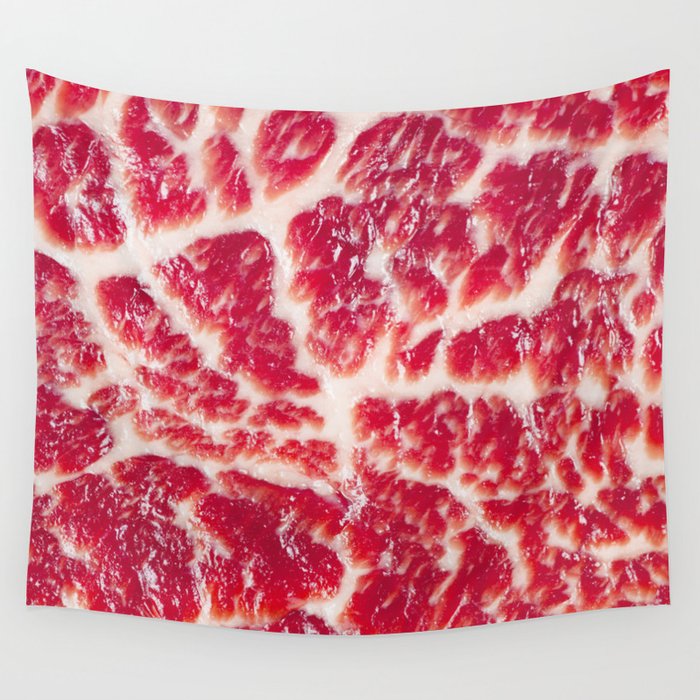The image depicts a highly realistic, close-up photograph of what appears to be a square slice of red meat, heavily marbled with white fat. The meat is presented in a way that it almost takes on an unnatural, artistic form, curving slightly and resembling a distorted shirt shape. The photograph, devoid of any other contextual elements, isolates the meat on a solid white background, reminiscent of a product image you might find in a marketing campaign for food items. The vivid colors, primarily dominated by the deep red of the meat interspersed with striking white fat, take center stage in the vertical rectangular frame, creating a stark and engrossing visual.